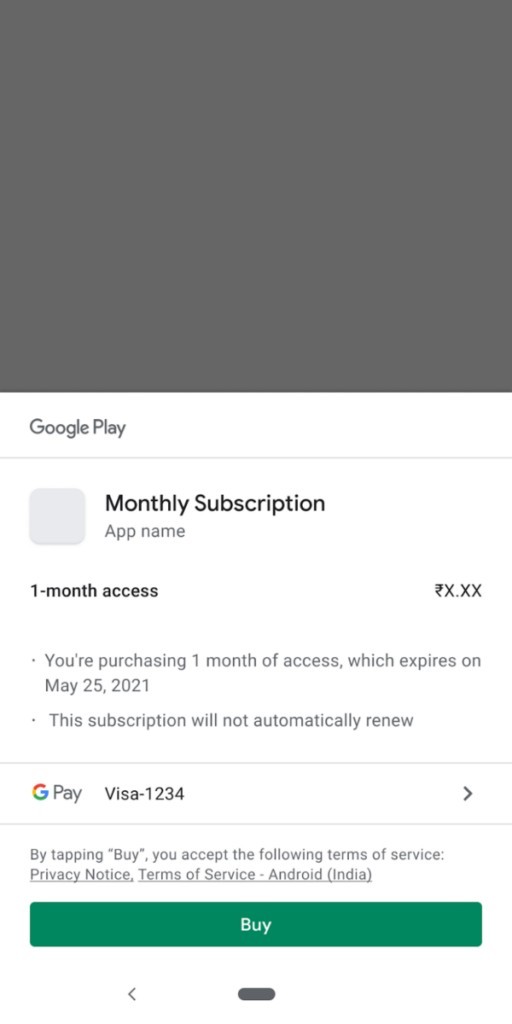The image is divided into two sections. The top portion features a plain gray square, while the bottom half is dominated by the Google Play logo. Beneath the logo, a label reads "Monthly Subscription," set against a muted grey background, with "app name" grayed out. This is followed by details for a one-month access subscription, displayed in black text on the left. On the right, there's a placeholder for the price, denoted by the Indian currency symbol (₹) and "X.xx."

The image notes that the subscription provides one month of access, expiring on May 25th, 2021, and explicitly states that the subscription will not renew automatically. Details of the payment method are given as "GPA Visa 134." By tapping the green "Buy" button, which features centered white text, users agree to the "Terms of Service" linked specifically for Android in India. At the bottom, typical UI elements of an Android device are visible, hinting that the screenshot was taken from such a device.